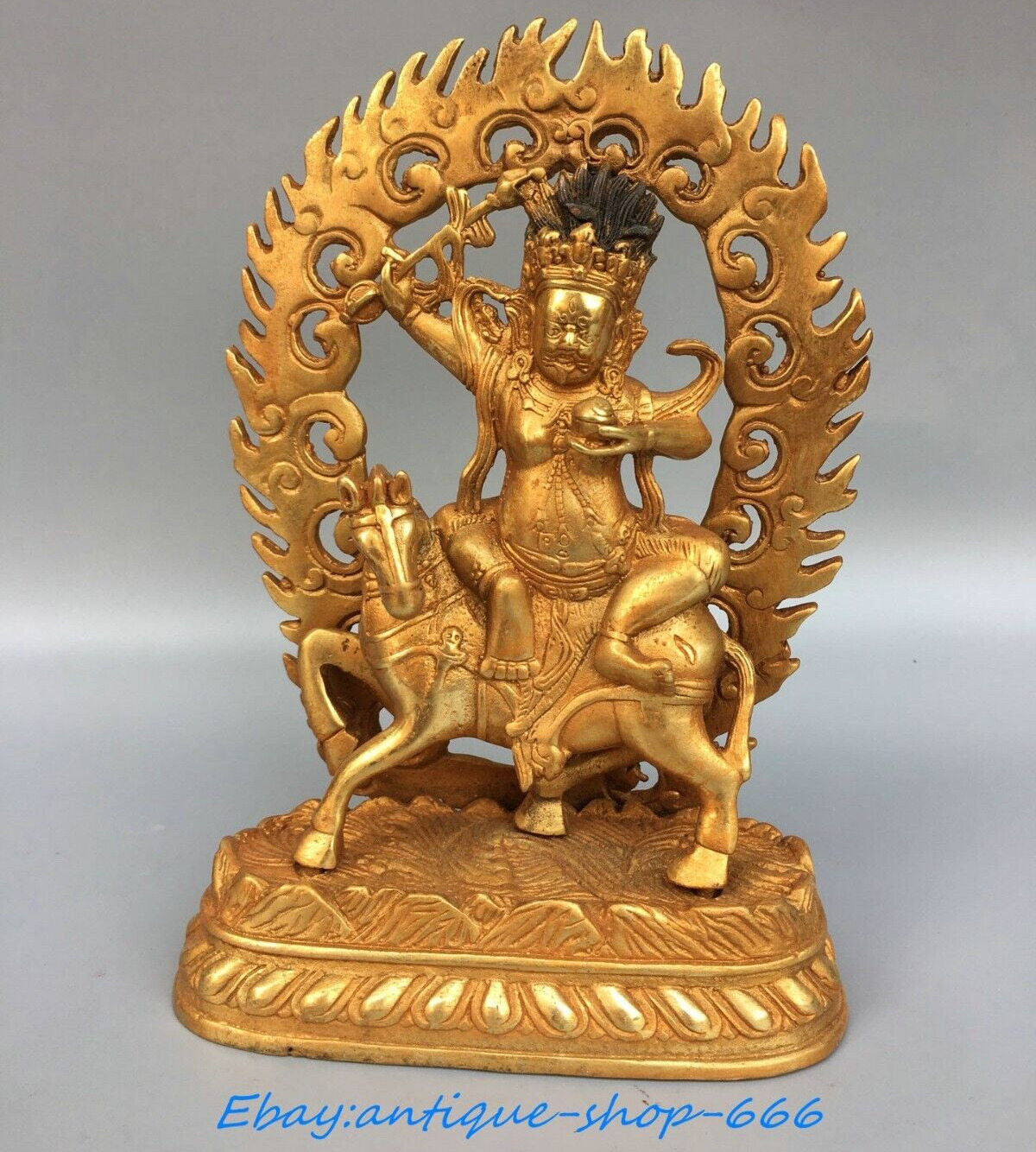In the image from an eBay listing, we see a detailed bronze statue of an Indian deity, possibly Hindu, seated sideways atop an intricately designed animal that resembles a cross between a wolf and a horse. The deity is adorned with a gold and black crown, which may have worn portions exposing the base material. He holds a ball in his left hand while steadying himself with his right, crouched within an elaborate arch that encircles and descends to the base of the statue, resembling divine flames or fire.

Set against a stark white background, indicative of a professional photoshoot, the sculpture rests on an ornate pedestal shaped like an oval flower bed, enhancing its vintage aesthetic. The listing details, written in blue cursive text on a gray backdrop below the statue, mention the eBay seller "eBay antique-shop.666," confirming its marketplace presence. The overall craftsmanship suggests a valuable antique piece, rich in cultural and religious significance.